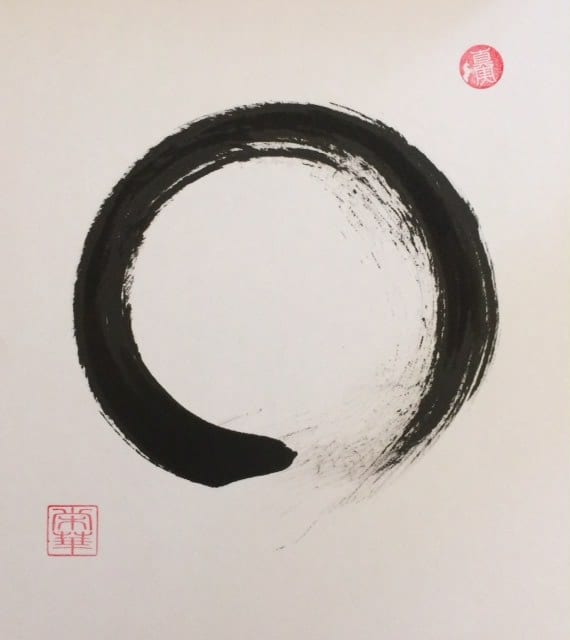The image depicts a painting on an off-white background, showcasing an incomplete black circle created with a single, counterclockwise brushstroke. Starting from the bottom right, the bold, paint-brushed line forms an almost complete circle but fades and distresses as it nears its origin, never fully connecting. The brushstroke, reminiscent of an upside-down snake, leaves intentional splashes and imperfections along the edges, adding a sense of dynamism and texture to the piece. Additionally, the painting features two stamps with characters in an East Asian script; one red circular stamp is positioned in the top right corner, while another red square stamp is located in the upper left corner.